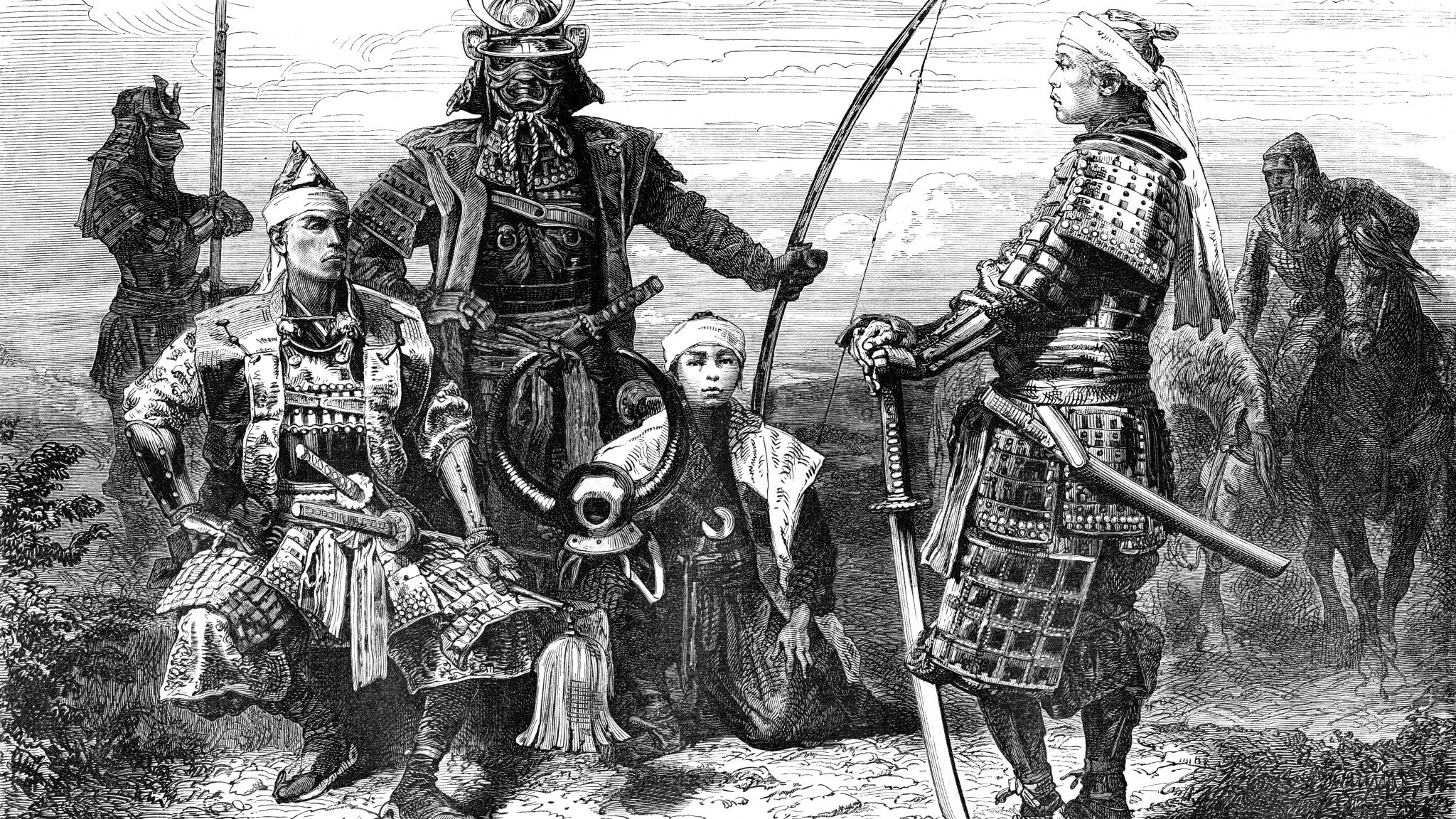This detailed black and white etching or pen and ink illustration depicts a scene with several Japanese samurai warriors in full, elaborately detailed armor, complete with metal plates and traditional weapons. At the forefront stands a man wearing a white bandana, resting his sword against the earth with both hands. To his left kneels a child in a robe, their demeanor poised and contemplative. Further left, a man stands elegantly, clutching a long bow and donning a large face mask and helmet, exuding a sense of readiness. Adjacent to him, a seated man with a pointed cap wrapped in a turban has two swords slung in his belt, contributing to the rich narrative of warriors prepared for engagement. A knight-like figure is observed to the left, contributing to the intricate interplay of characters. The right side of the scene features a mounted samurai, adding a dynamic element to the otherwise still tableau. The entire composition is highly intricate, with varying shades of gray, intricately etched details, and scenic outdoor elements, likely capturing a moment of strategic preparation or solemn reflection before a battle.